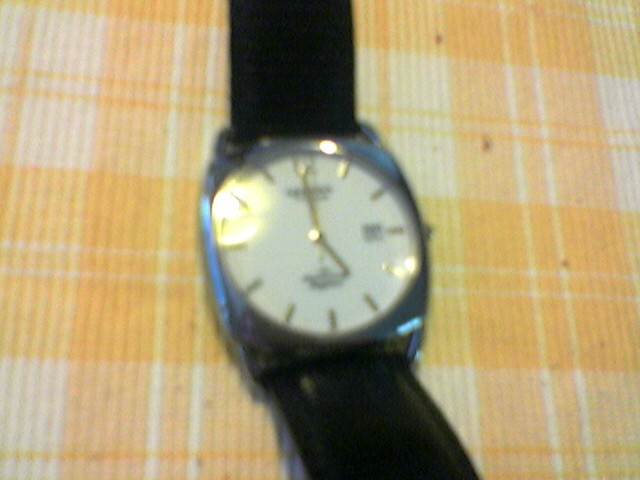This detailed, color photograph captures a close-up of an elegant watch face. The image is somewhat blurred, with notable light reflections on the left side, making it challenging to discern finer details. The watch boasts a round face framed by a slightly squared band, featuring metallic edges that add a touch of sophistication.

Though exact numbers are indiscernible, the indices appear to be golden markers. The gold hands indicate the time as 5:00, aligning precisely at the 12 and 5 positions, with no visible second hand. There's notable text just beneath where the 12 would conventionally be and above where the 6 would reside.

Adjacent to the presumed 3-o'clock marker, there's a smaller panel, potentially a date window, though the blur obscures specific information. The watch is accentuated by a sleek black band attached to the top and bottom.

The timepiece is set against a vibrant surface adorned with an orange and white check pattern, enhancing the overall aesthetics of the photograph.